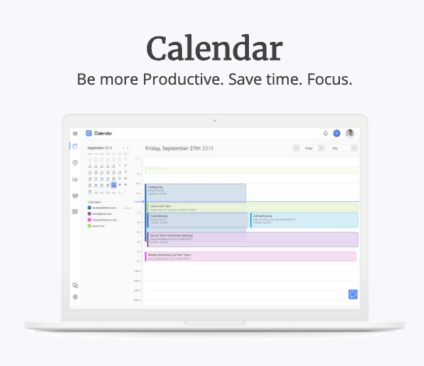This is an advertisement with a clean, off-white background. The ad is a small square shape, dominated by bold black text at the upper center reading "CALENDAR." Below this, in smaller black font, is the phrase "B-MORE-PRODUCTIVE," with an improperly capitalized "P." Following are the phrases "save time," "focus," each punctuated by periods.

Beneath the text, a graphic of an open white laptop is prominently displayed. The laptop features white bezels, and its screen shows a calendar application. Although the specific software cannot be identified due to the small size of the ad, the calendar layout is clear. On the left side of the screen, a calendar grid is visible, and on the right side, there is an area for adding appointments.